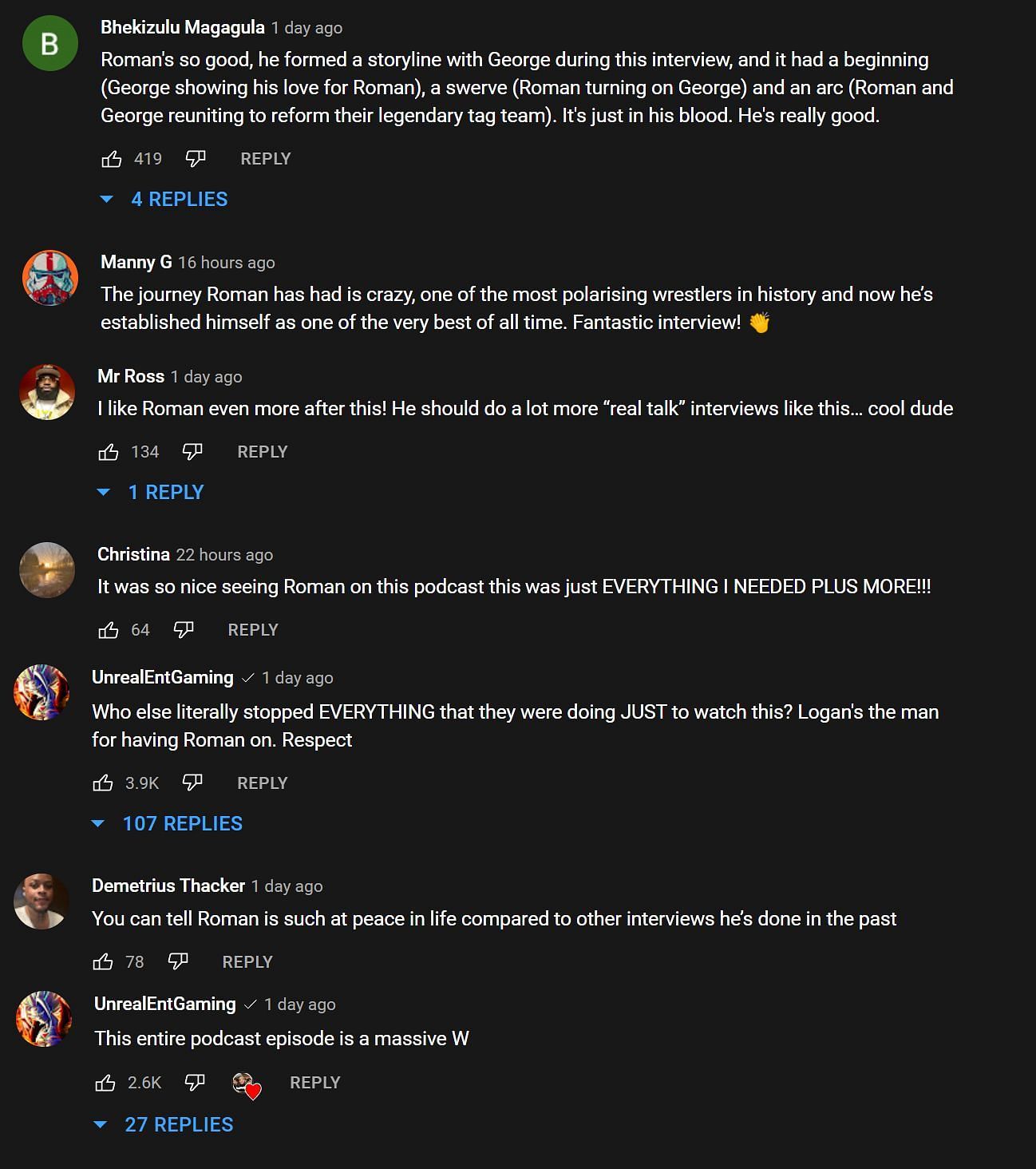Against a black background, user comments praising Roman’s interview are displayed:

1. **BHEKEKIZULU MAGAGULA, one day ago:** "Roman's so good. He formed a storyline with George during this interview, starting with George showing his love for Roman. There was a swerve where Roman turned on George, creating an arc that led to Roman and George reuniting to reform their legendary tag team. This is just in his blood. He's really good."
   - **Likes:** 419 
   - **Replies:** 4 (View Replies)

2. **Manny G, 16 hours ago:** "The journey Roman has had is crazy. One of the most paralyzing wrestlers in history, now he's established himself as one of the very best of all time. Fantastic interview."
   - **Likes:** Not specified

3. **Mr. Ross, one day ago:** "I like Roman even more after this. He should do a lot more real talk interviews like this. Cool dude."
   - **Likes:** 134
   - **Reply:** 1 (View Reply)

4. **Christina, 22 hours ago:** "Yes, it was so nice seeing Roman on this podcast. This was just everything we needed plus more."
   - **Likes:** 64

5. **Unreal ENT Gaming, one day ago:** "Who else literally stopped everything they were doing just to watch this? Logan is the man for having Roman on. Respect."
   - **Likes:** Not specified